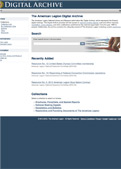The image is a heavily blurred and highly compressed screenshot of a website page titled "Digital Archive." The screenshot is not only blurry but also very small and has been cropped, removing key elements like the logo and portions of the navigation menu on the left. The visible but illegible navigation menu is positioned on the left side of the page. On the right, there are about four categories with bolded titles, a search bar function, and various text descriptions, none of which can be read due to the image's poor quality. The website features a large blue banner at the bottom and a thinner blue banner at the top.